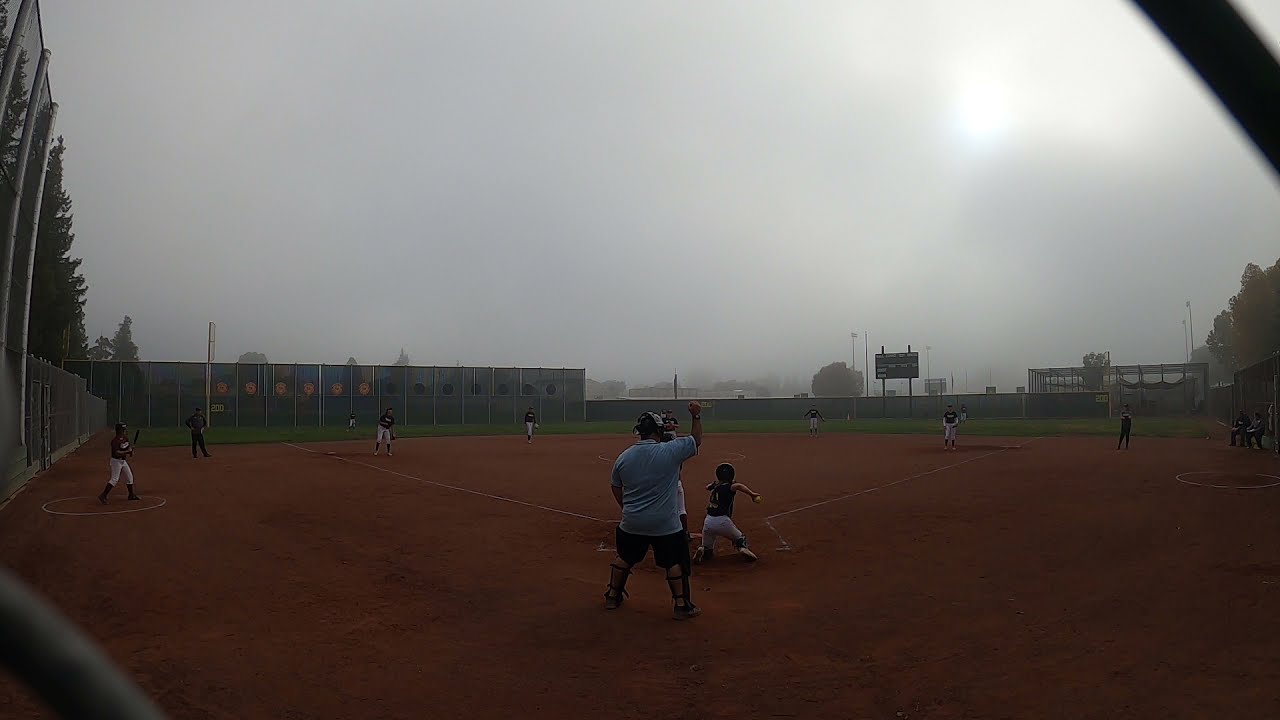In this image of a youth baseball game, you see young children, likely between 10 to 13 years old, actively participating on a dirt field lined with white boundary markings. A striking figure in the center is the umpire, dressed in a blue shirt and protective gear, signaling a strike with his closed fist raised in the air. To his side stands a small child ready to bat, while other kids are positioned at first base, shortstop, and third base. The catcher, dressed in traditional baseball attire, is prepared to throw the ball. Surrounding the field, a black scoreboard is visible alongside a fence encircling the area, with a few spectators watching from the sidelines. The backdrop contains buildings and trees, all under a mostly gray, cloudy sky with the sun faintly piercing through. The overall scene is bathed in the soft, diffused light of a gloomy day.